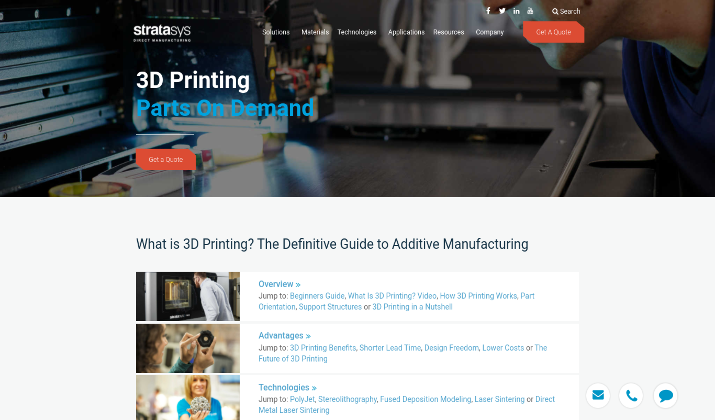The screenshot showcases the Stratasys company's website, which specializes in the 3D printing market, offering 3D printing models, parts, and other related products. In the top half of the image, the background features a 3D printer with a person's face visible to the right, looking at the printer. Overlaying this background, in the top left corner, the Stratasys company name appears in white text, followed by the headline "3D Printing" in white, "Parts on Demand" in blue, and an orange box with white text instructing, "Get a Quote." Clicking this box redirects users to a webpage for obtaining a quote on desired products.

Centrally positioned on the top section is a horizontal navigation bar with links to sections such as Solutions, Materials, Applications, and others, offering detailed information about the company's products.

The bottom half of the screenshot features a white background with the headline "What is 3D Printing? The Definitive Guide to Additive Manufacturing" in black text. Below this, there are clickable links leading to different sections of the website, such as an Overview, Advantages, and Technologies. Each link is accompanied by small images: one of a person looking at a 3D printer, another holding a 3D-printed object, and a woman displaying another 3D-printed item. These images visually enhance the page and provide insights into the capabilities and applications of 3D printing by Stratasys.